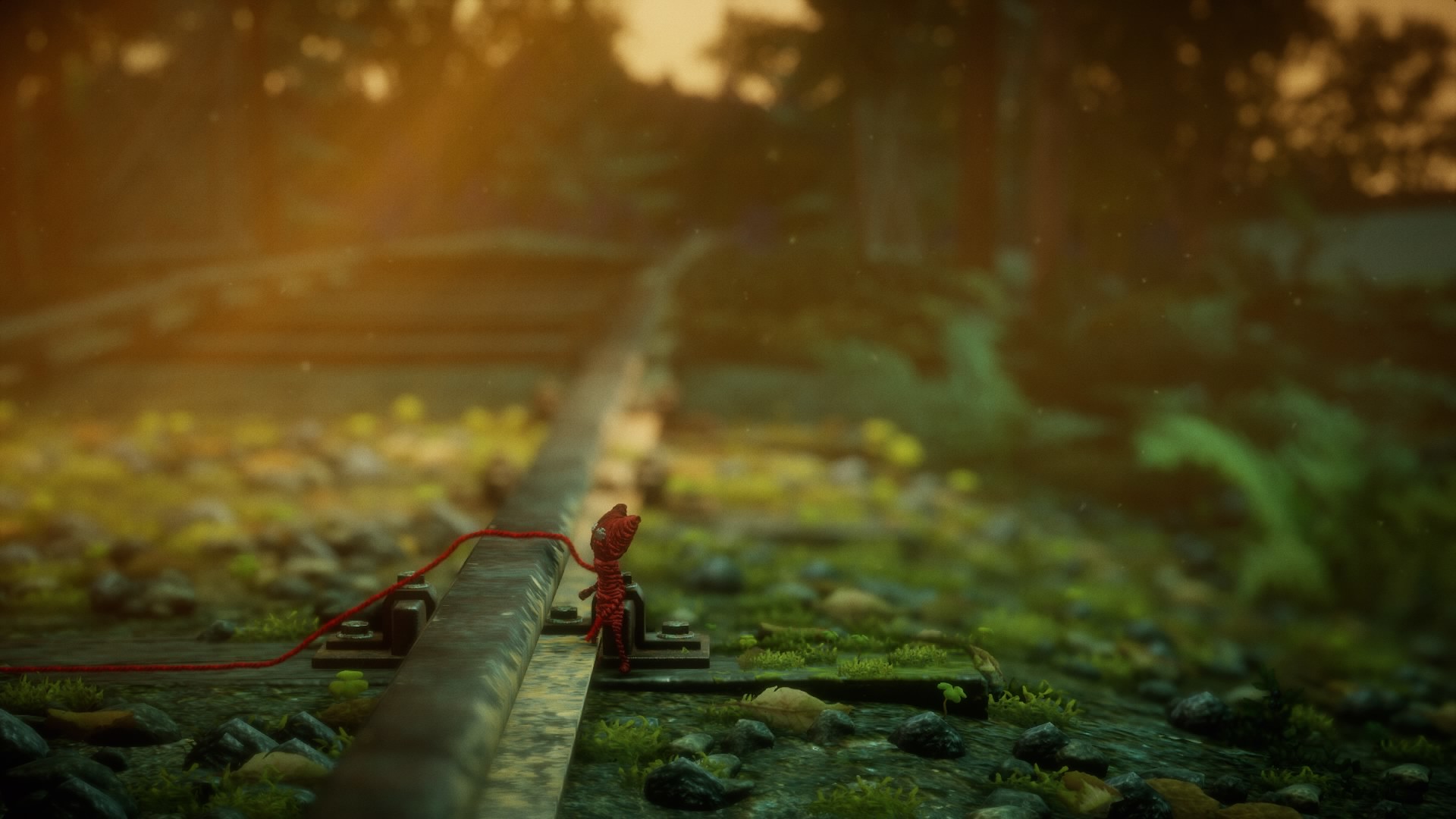A captivating image captures a unique ground-level perspective of a train track, where the focus is on the right-side rail. In the foreground, a charmingly crafted knit figure made of red yarn, resembling a cat or a small person with ears atop its head, sits prominently. The yarn appears to be unraveling and trails off to the left side of the frame. The surrounding environment is richly detailed, with an array of gravel, leaves, and patches of moss vividly visible. Soft sunlight peeks through, suggesting either dawn or dusk, casting a gentle glow along the center of the track and filtering through the trees in the background. The overall atmosphere of the image is dark and moody, enhanced by the interplay of light and shadow.